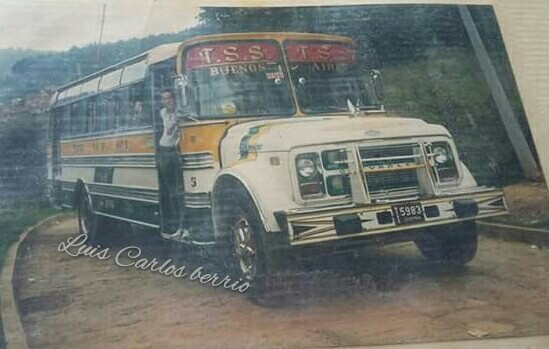This image depicts a vintage school bus, potentially captured in an old and blurry photograph or as a painted mural on a wall, with bricks or corrugated cardboard possibly visible in the background. The bus, primarily white with a striking yellow stripe running along its middle, features a distinctive front marked by a red stripe above the windows and a black stripe below. The hood displays the name "TSS" in Buenos, suggesting a South American origin, likely Argentina, with the artist or owner, "Luis Carlos Berrios," or alternatively "Berrie," elegantly inscribed below. The bus's design includes gold letters spelling out "TSS" on the front and side windows, and it sports a unique winged hood ornament. The license plate reads "5993." The bus appears to be stationary on a road that could be dirt, stone, or concrete, with a visible curved curb. Surrounding the bus, dense greenery with trees and bushes forms the backdrop, contributing to the overall rustic and historical feel of the scene. A person can be seen standing in the open doorway on the right side of the vehicle, adding a human element to this intriguing tableau.